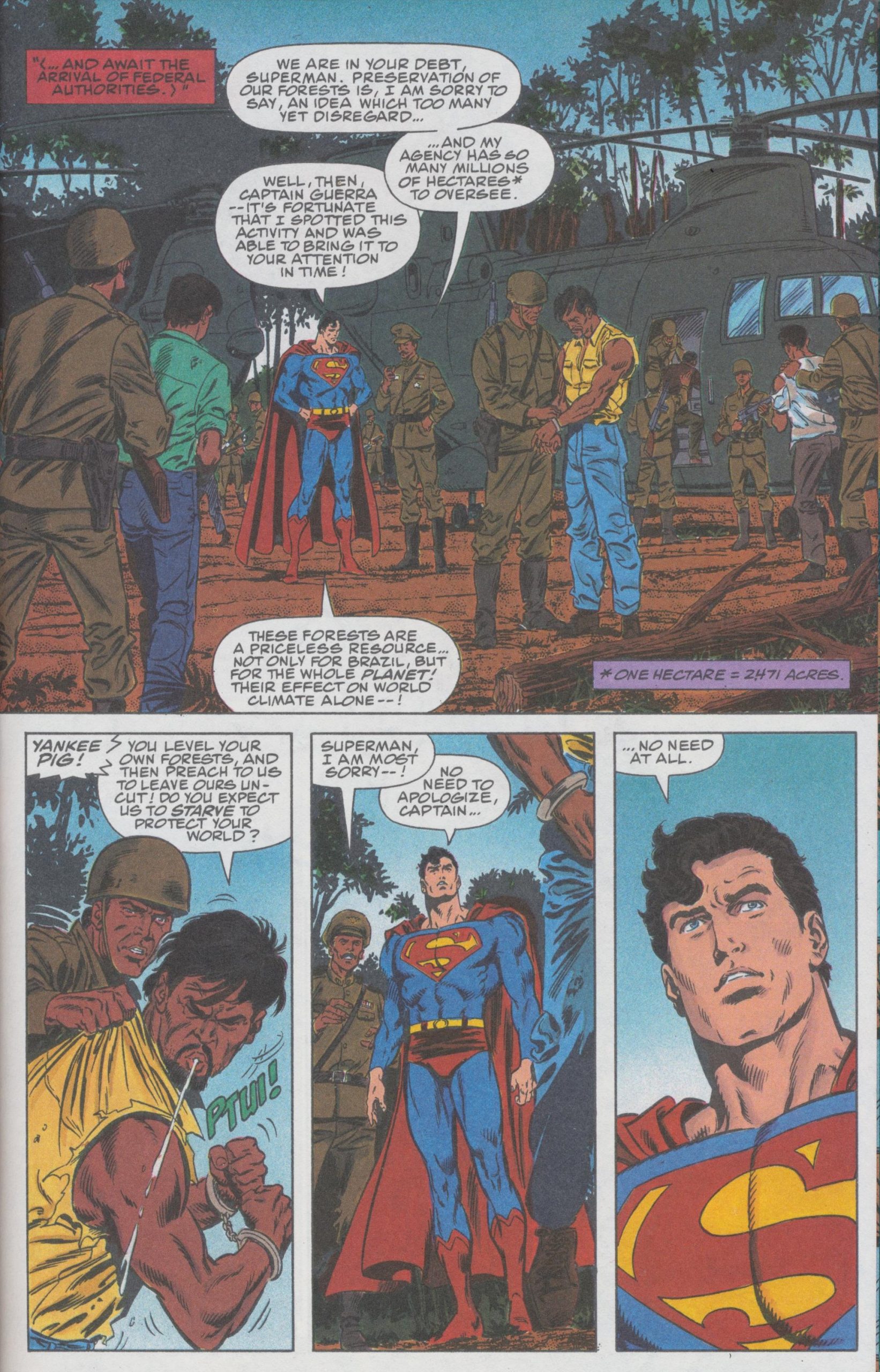This detailed, full-page portrait orientation comic book scene captures Superman in action. At the top half of the page, Superman stands slightly left of center, conversing with several soldiers. They are assisting imprisoned or injured people, reflecting the storyline's focus on forest preservation. White dialogue balloons with black text fill the scene, including one where a character says, "We're in your debt, Superman. Preservation of our forests is, I'm sorry to say, an idea which many yet disregard. My agency has millions of hectares to oversee."

A gray army helicopter rests on the right side, poised for transporting people, framed by woods in the background. Below this are three additional comic panels: 

1. The first panel features a soldier arresting a spitting felon.
2. The second panel centers on Superman responding, “It’s fortunate that I spotted this activity and was able to bring it to your attention in time.”
3. The third panel reinforces the theme, with Superman emphasizing, "These forests are a priceless resource not only for Brazil but for the whole planet. Their effect on the world climate alone…”

In vivid color illustration consistent with classic comic book style, the characters wear various uniforms, with Superman’s iconic costume prominent against the lush green and muted tones of the forest. A purple rectangular panel explains, "One hectare equals 2.471 acres," emphasizing the scale of the environmental stakes involved. The page is visually dynamic with shades of blue, yellow, gray, white, and purple, ensuring the story's message is clearly conveyed.